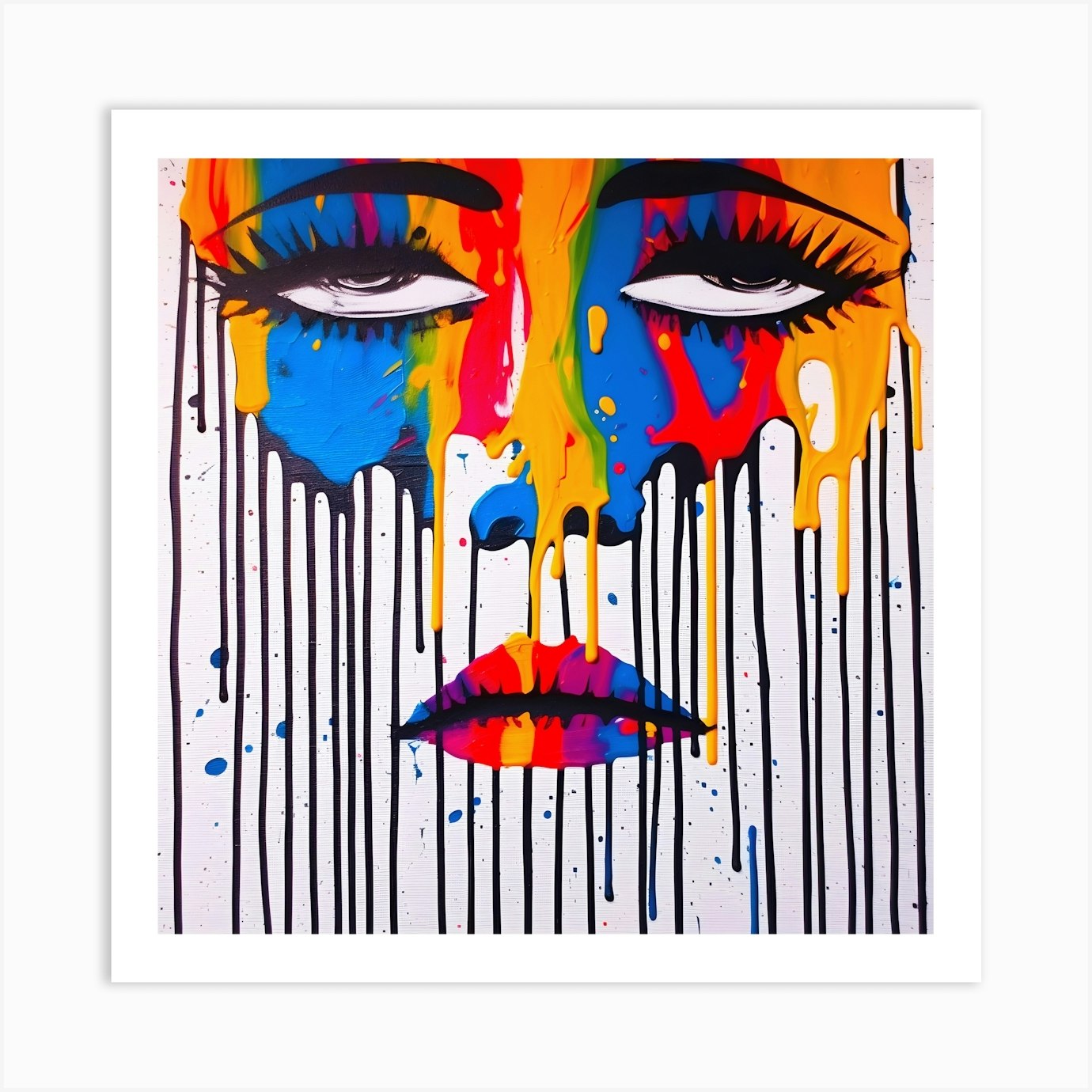This artwork is a modern, high-end painting set within a perfectly square white frame, featuring two white borders. The piece portrays an abstract yet identifiable face of a woman against a white background. Her sorrowful eyes, framed by thick, carefully groomed black eyebrows and long eyelashes, gaze upwards. The eyes themselves are a striking combination of black and white. The woman’s nose, mainly blue with splashes of yellow paint, merges into vibrant multicolored lips, which display a gradient of blue, purple, red, yellow, and orange hues, separated by a distinct black line.

Vertical streaks of paint descend from her forehead to below her nose, almost resembling teardrops, perhaps symbolizing sorrow. These streaks incorporate a vivid range of colors, including yellow, red, blue, orange, and green, which intermingle with numerous black paint drips, contributing to the melancholic expression. The absence of a defined jawline further emphasizes the fragmented, emotional nature of the image. The piece’s intricate play of colors and emotional depth is accentuated by the notable absence of any text, words, or numbers, allowing the visual elements to speak powerfully on their own.